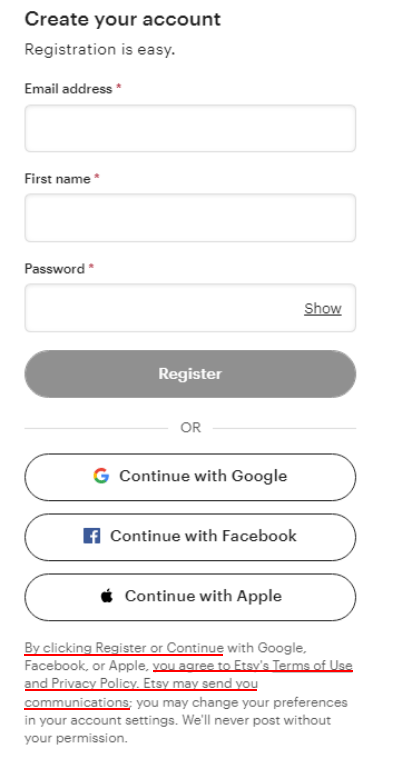Screenshot depicting an account creation page with a clean and minimalistic design. The background is stark white with centrally positioned black text headers guiding the user through the registration process. 

At the top, bold text reads "Create Your Account" followed by a subheader declaring, "Registration is easy." Below this, there are several fields with accompanying red asterisks indicating required information:
1. "Email Address" with a white input box.
2. "First Name" with a white input box.
3. "Password" with a white input box and a gray "Show" option beside it.

Underneath these inputs, a large gray box labeled "Register" with white text is prominently displayed. 

Beneath the "Register" button, the word "or" is written in black. Following this, there are three additional options for registration, each within a white box adorned with icons and text representing various third-party services:
1. "Continue with Google," highlighted by the red, gold, green, and blue Google icon.
2. "Continue with Facebook," distinguished by a blue background and a white "F" logo.
3. "Continue with Apple," marked with a black Apple icon.

At the bottom, there is a statement in gray text regarding the site's terms and conditions. Part of this statement is underlined in red for emphasis: "By clicking register or continue with Google, Facebook, or Apple, you agree to Etsy's terms of use and privacy policy. Etsy may send you communications. You may change your preferences in your account settings. Will never post without your permission."

Overall, the image quality is excellent with clear, readable fonts, and devoid of pixelation, blurring, or any extraneous objects.